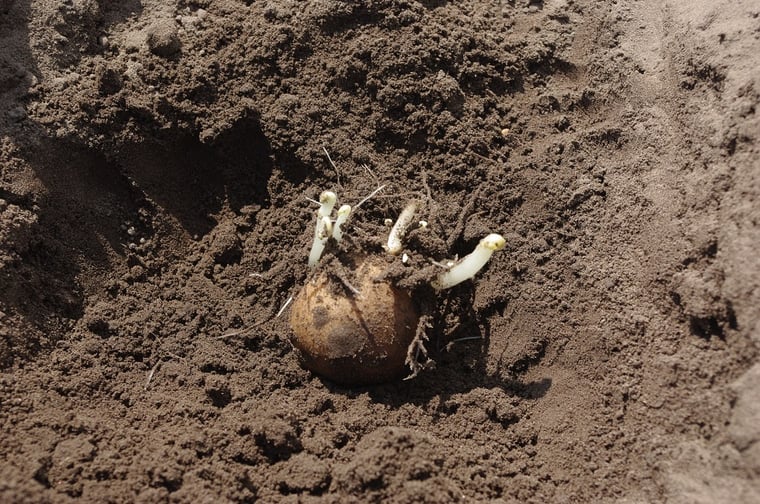The image captures a close-up, top-down view of a single potato that has recently been excavated from the soil. This potato, which resembles a sea potato or possibly a russet, appears golden brown beneath its network of roots. The soil surrounding the potato shows variations in moisture: dry on the right side, while almost black and moist in the middle. Prominent white roots, some large and thick, emerge from five significant "eyes" on the potato, with skinnier roots extending from the sides. The scene, taken during the daytime, reveals a well-defined contrast between the dark, rich earth and the lighter hue of the potato, which sits partially buried and ready for planting.